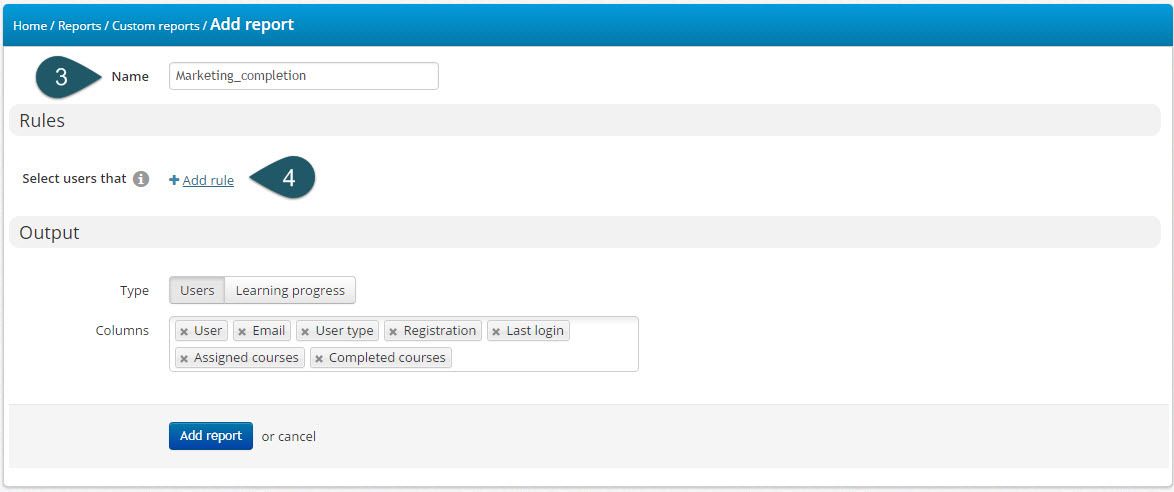The image depicts a detailed interface layout, likely from a software tool used for generating custom reports. At the top is a long blue header featuring a breadcrumb path in white text: "Home / Reports / Custom Reports / Ad Report." "Ad Report" is bolded for emphasis.

Below the header, a section begins with a teal teardrop icon pointing right with the number "3" in white, directing attention to the word "Name," which is written in black. Adjacent to this is an input box with a white background and gray text that reads "marketing_completion."

Further down is a long, rounded rectangle labeled "Rules" in dark gray. Below this, there’s a label "Select Users" accompanied by a gray circle with a white 'i' (information icon) and a greenish plus sign labeled "Add a Rule."

Another teal teardrop icon, this time with the number "4" in white and pointing left, highlights the label "Output," which is contained within another long, rounded rectangle. 

Under the "Output" section, the word "Type" appears in gray next to a small gray square labeled "Users" (USERS). Accompanying this is a long rectangle indicating "Learning Progress." 

Following this is a "Columns" section with a white background. Inside the rectangle are multiple labels in gray text, each followed by a small 'X' for removal: "User," "Email," "User Type," "Registration," "Last Login," "Assigned Courses," and "Completion Courses."

Finally, at the bottom is a long gray rectangle and a prominent blue button labeled "Add Report" in white text, alongside a gray "Cancel" option.

This comprehensive caption covers the intricate details and organizational layout of the interface elements depicted in the image.